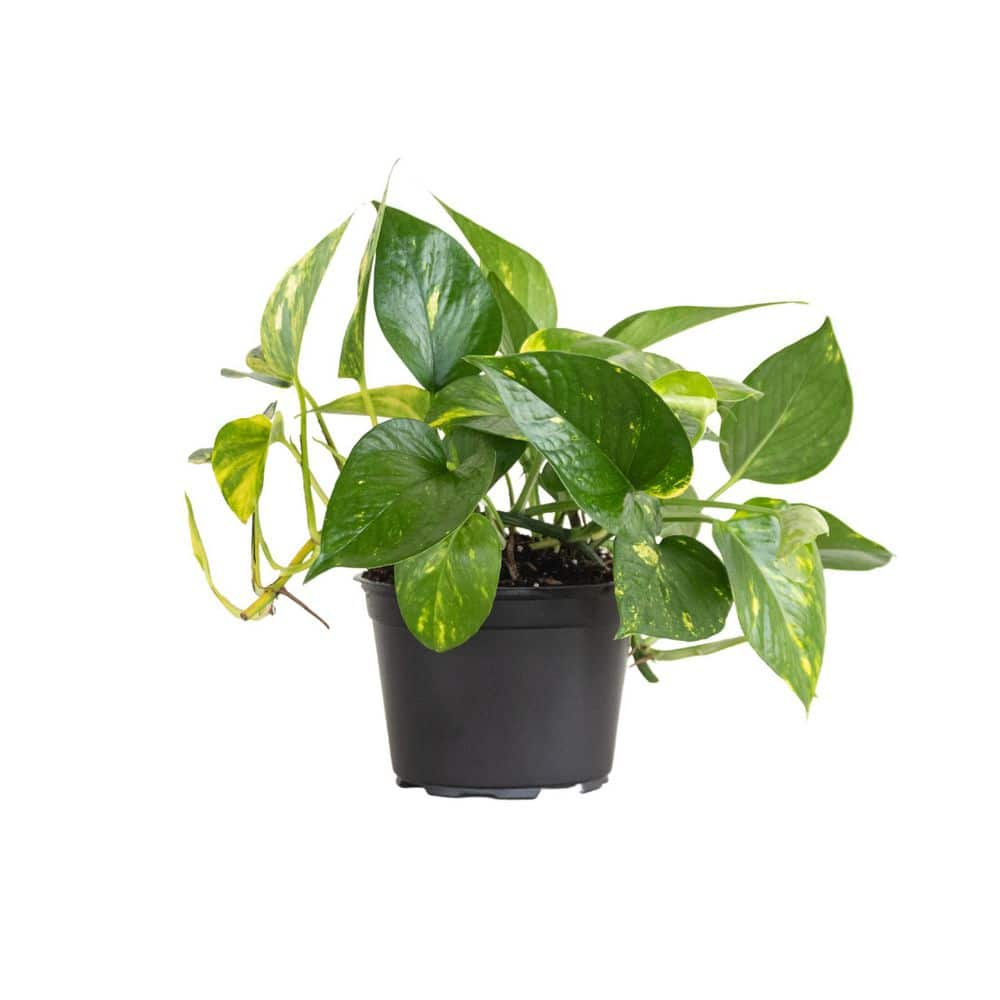This detailed photograph features a healthy, young philodendron potted in a small black plastic pot, possibly a pint or a quart in size, and filled with dark brown soil flecked with white fertilizer spots. The philodendron, with approximately 20 leaves and four or five branches, is vibrant and varied, showcasing predominantly green, glossy leaves accented with yellow spots and chartreuse tips. Despite its youth, the plant has abundant new growth and stands very upright; none of its vines trail down, suggesting it has been recently trimmed. The pot reveals visible roots growing out from the bottom, indicating a robust root system. The plant is staged against a clean white background, implying that the image could be intended for online plant sales, highlighting its pristine condition and suitability for potential buyers looking to repot it or use it as an office plant.